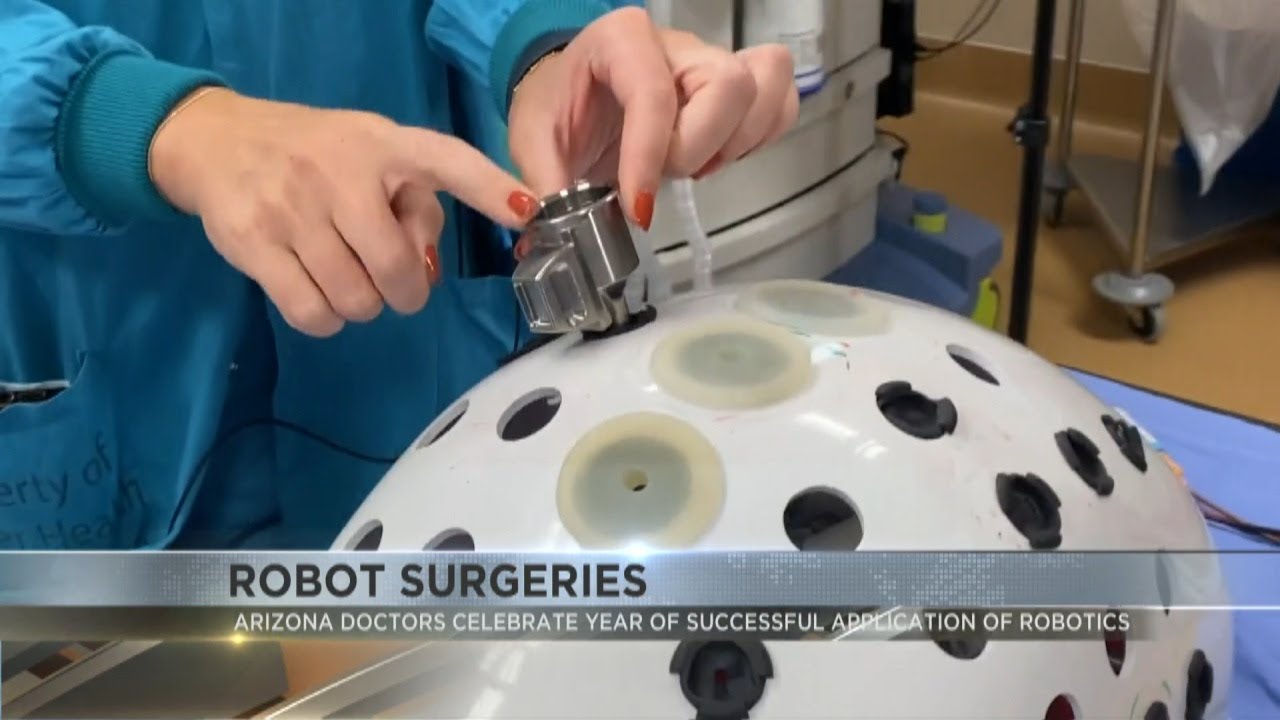In this photorealistic image, we observe a close-up of a person in the upper left corner, identifiable only by their hands adorned with red nail polish and clad in blue surgical garb. They are working with a silver cylindrical device, which they are attaching to a domed, white, shiny plastic object featuring several drilled holes. The scene clearly indicates a medical environment, emphasized by various medical devices and stands in the background, while a blue surgical drape supports the domed object. A news-style banner at the bottom of the image reads: "Robot Surgeries," followed by "Arizona Doctors Celebrate Years of Successful Application of Robotics," implying this is a screenshot from a TV news broadcast celebrating the achievements of robotic surgery in Arizona.